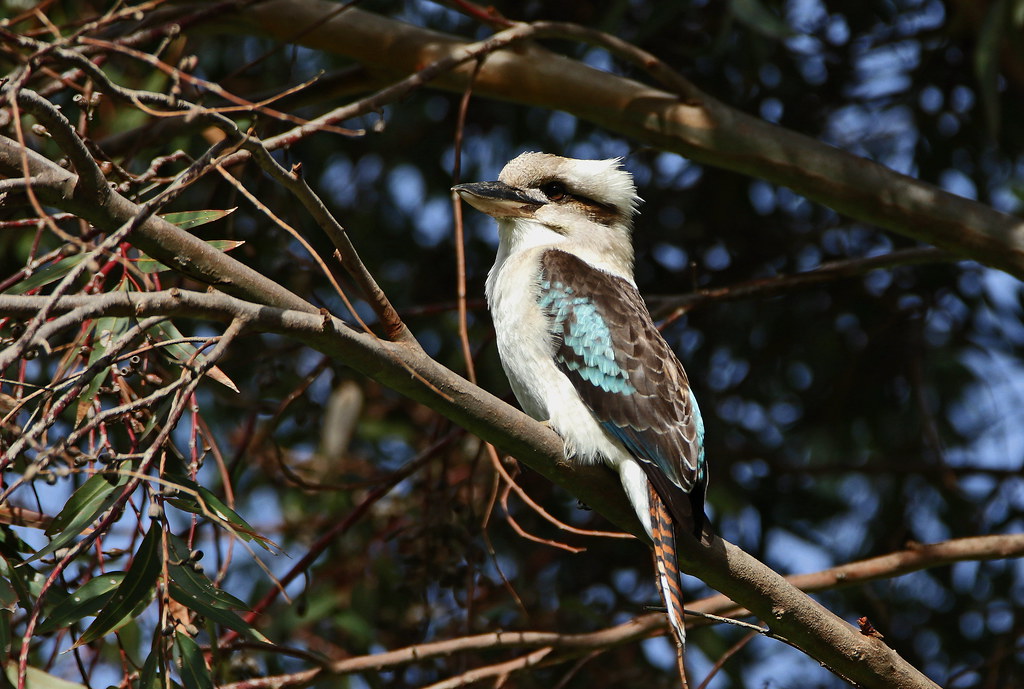This close-up photograph features a small bird, approximately three to four inches tall, perched on a tree branch. The branch has long, green leaves with some red stems, though the tree itself appears to be dying, bereft of foliage except in small sections. The bird, which looks somewhat disheveled as though it has bedhead, has a distinct coloration: its body is predominantly white with a brown lower beak and a black upper beak. Its eyes are dark brown, and it has a black stripe that extends from around its eye to the back of its head. The bird's wings are gray, accented with patches of light blue in the middle and outer edges, and the tips are black. Its long, slender tail feather is strikingly striped with black and orange. One partially visible claw is yellowish. The background reveals a blurred blue sky, indicating the photo was taken during the day. The bird is looking off to the left side of the image, adding a contemplative feel to the scene.